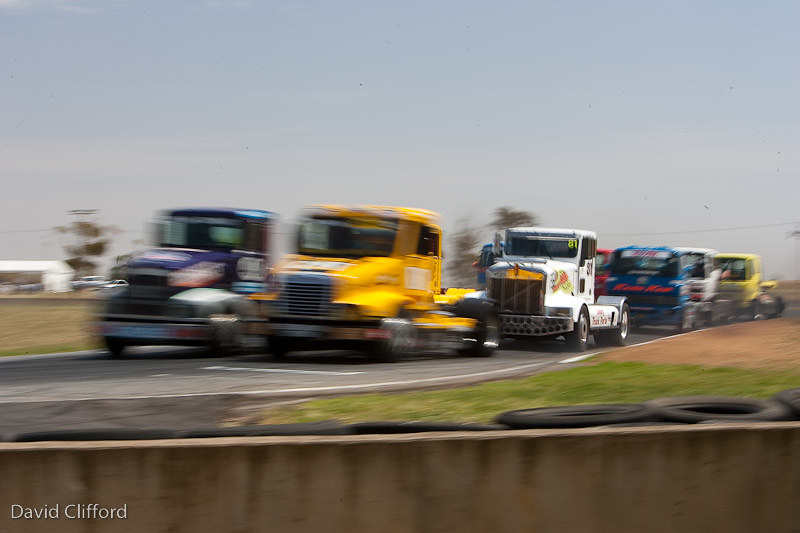This color photograph, taken outdoors during the daytime, captures the intense motion of a semi-truck race on a racetrack. The image predominantly features several truck cabs without trailers, speeding closely together, creating a blurred effect, especially on the leading vehicles. In the foreground, the yellow and dark blue trucks are the blurriest, indicative of their high speed or slight out-of-focus capture. Trailing these are a white truck, followed by additional trucks in various colors including blue, white, purple, yellow, and red, though the exact sequence and clarity diminish towards the back due to the blur and obstructions from leading trucks.

The racetrack is an asphalt path bordered by a concrete retaining wall marked with dark stains possibly from liquid runoff. In front of this wall, there are stacks of black tires. Surrounding the track are patches of green grass and brown dirt. In the background, a somewhat obscured tan building with a white roof stands adjacent to a tall tree with lush, green foliage. The sky above is gray, hinting at overcast weather conditions. The photograph credits “David Clifford” are noted in white font at the bottom left-hand corner. Overall, the dynamic scene suggests the thrill and velocity of the race.